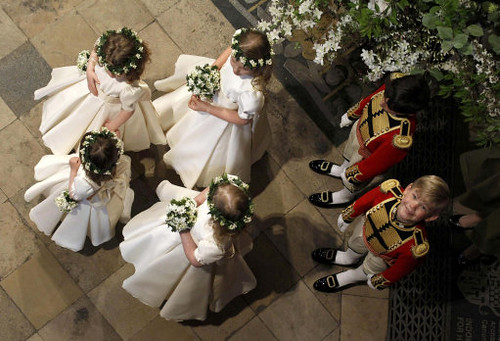This color photo, taken from above, captures a charming scene indoors, presumably part of a royal wedding. Six children are assembled on what appears to be a tiled cement area. In the front row, four little girls are dressed in elegant, creamy white dresses with crinolines, giving them a full, pleated appearance. Each girl wears a delicate wreath of white flowers and green leaves, almost like halos, atop their heads, and they hold matching bouquets of white flowers.

Behind them stand two little boys in elaborate, military-style outfits reminiscent of the palace guard uniforms. The boys' attire includes striking red jackets adorned with black and gold epaulettes, black and gold cuffs, and a black chest plate with gold accents. Their outfits are completed with white stockings and black patent loafers featuring gold buckles. One boy has dark hair, and the other, a blonde, is smiling up at the camera. The scene has an air of anticipation, as the children patiently await their turn, likely to walk down the aisle.